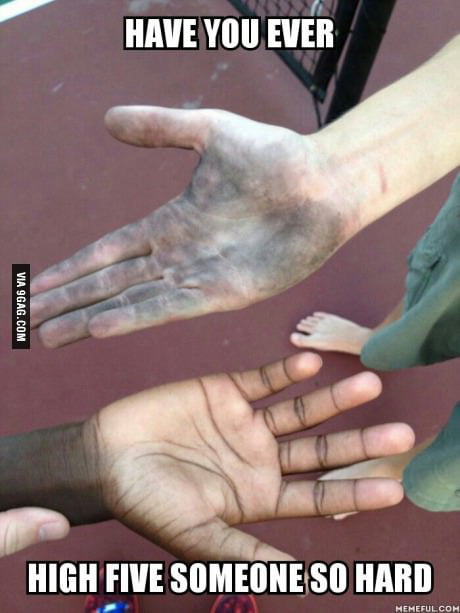This meme features a humorous "top text, bottom text" format with the VN9GAG watermark positioned on the left-hand side. The meme asks, "Have you ever high-fived someone so hard?" The background image displays two outstretched forearms, one belonging to a white person (above) and the other to a Black person (below). The Black individual's palm, which is naturally a lighter shade, is humorously depicted as being covered in soot, suggesting they have transferred black pigment onto the white person's hand through the high-five. This visual joke plays on the exaggerated idea that the high-five was so intense it caused their skin colors to transfer, reflecting a playful and hyperbolic take on physical interaction.